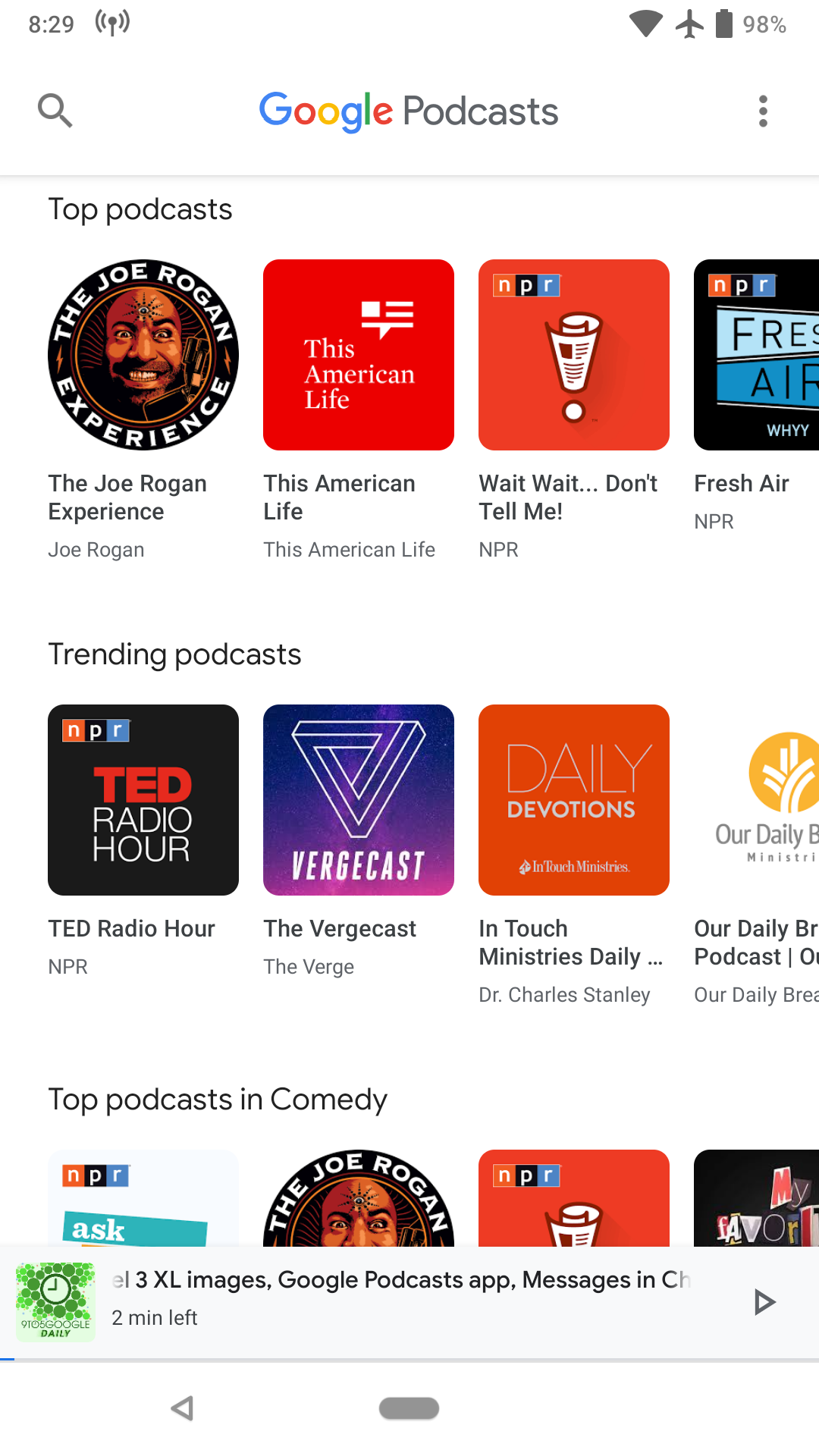Screenshot of a smartphone displaying the Google Podcasts app with various details. The time on the phone is 8:29, and the battery is at 98%, indicating plenty of power. In the Google Podcasts app, trending and top podcasts are displayed. The featured podcasts include "The Joe Rogan Experience," which has a Klingon visual element, "This American Life," "Wait Wait... Don't Tell Me!" from NPR, "Fresh Air" also from NPR, "TED Radio Hour," "The Vergecast," "In Touch Ministries" with Charles Stanley, and "Our Daily Bread Podcast."

In the comedy category, "The Joe Rogan Experience" is again listed alongside "Wait Wait... Don't Tell Me!" and several other cut-off entries, including one that partially reads "My Save." A notable green logo with a clock icon is present, though the text associated with it is partially obscured, making it unreadable. It mentions "Google Podcasts" in the context of apps and includes references to messages in the Chromebook, with a note indicating approximately two minutes remaining. The screenshot captures a comprehensive view of the user's Google Podcasts interface and system status at the time.